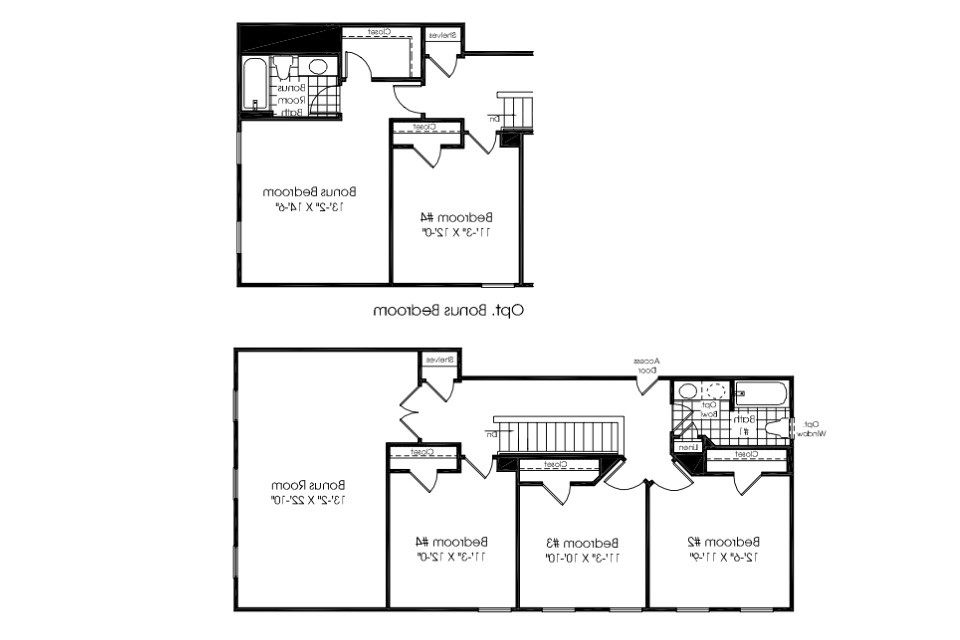This image features a detailed floor plan of a house, partitioned into two sections. The top section illustrates an area containing Bedroom 4 and a Bonus Bedroom. Despite being reversed, making the text challenging to read, certain key details are distinguishable. The Bonus Bedroom is highlighted by two windows and an ensuite bathroom, complete with a closet and a doorway. Adjacent to Bedroom 4, a staircase leads out, further connecting to the main level.

Descending to the primary house layout in the lower section, the Bonus Bedroom and its two windows are reiterated, alongside Bedroom 4. Clear delineations of doorways and closets are evident, marking the transitions between different rooms. Bedroom 4 connects seamlessly to Bedrooms 3 and 2, each equipped with built-in closets.

The plan also showcases the staircase’s full length, which links to an entrance at the front. A detailed bathroom area is illustrated, consisting of a bathtub, shower, handwashing basin, and tiled flooring. This bathroom services Bedrooms 2 and 3, with doorways that uniquely align against a single wall, offering a distinct architectural feature.